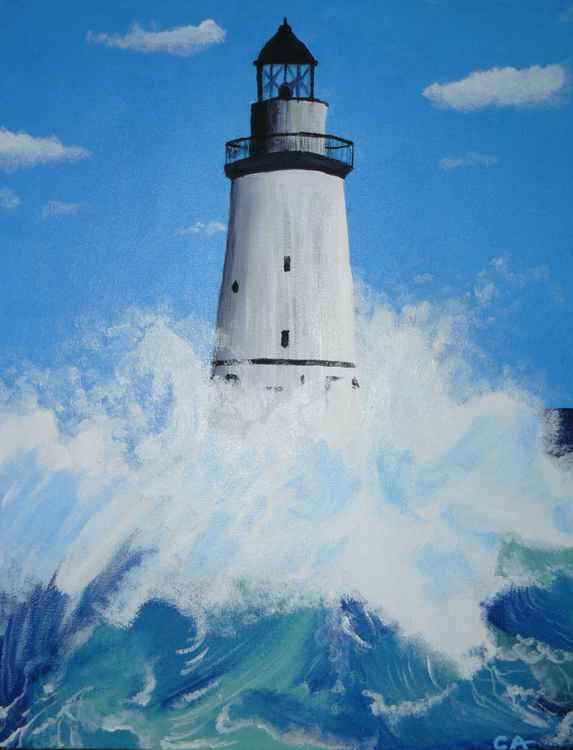This watercolor painting depicts a tall, traditional lighthouse standing at the center of the image, surrounded by turbulent waves crashing violently against its base. The towering structure is predominantly white with a gray hue, featuring a black observation deck and a black roof. At the top, enclosed in glass, sits a light source likely used to guide mariners. The sky above is a light blue, adorned with scattered clouds, creating a stark contrast against the deep blue ocean below. The sea is animated with vigorous waves, characterized by white sea foam and bubbles, indicating a powerful high tide assaulting the lighthouse. Despite the commotion in the water, it's evident that the painting does not depict rain, but instead a scene of natural marine turmoil. The horizon line is almost obscured by the aggressive waves, further emphasizing the lighthouse's battle against the relentless sea. A subtle detail includes the artist's signature, "CA," in light blue at the bottom right of the painting.